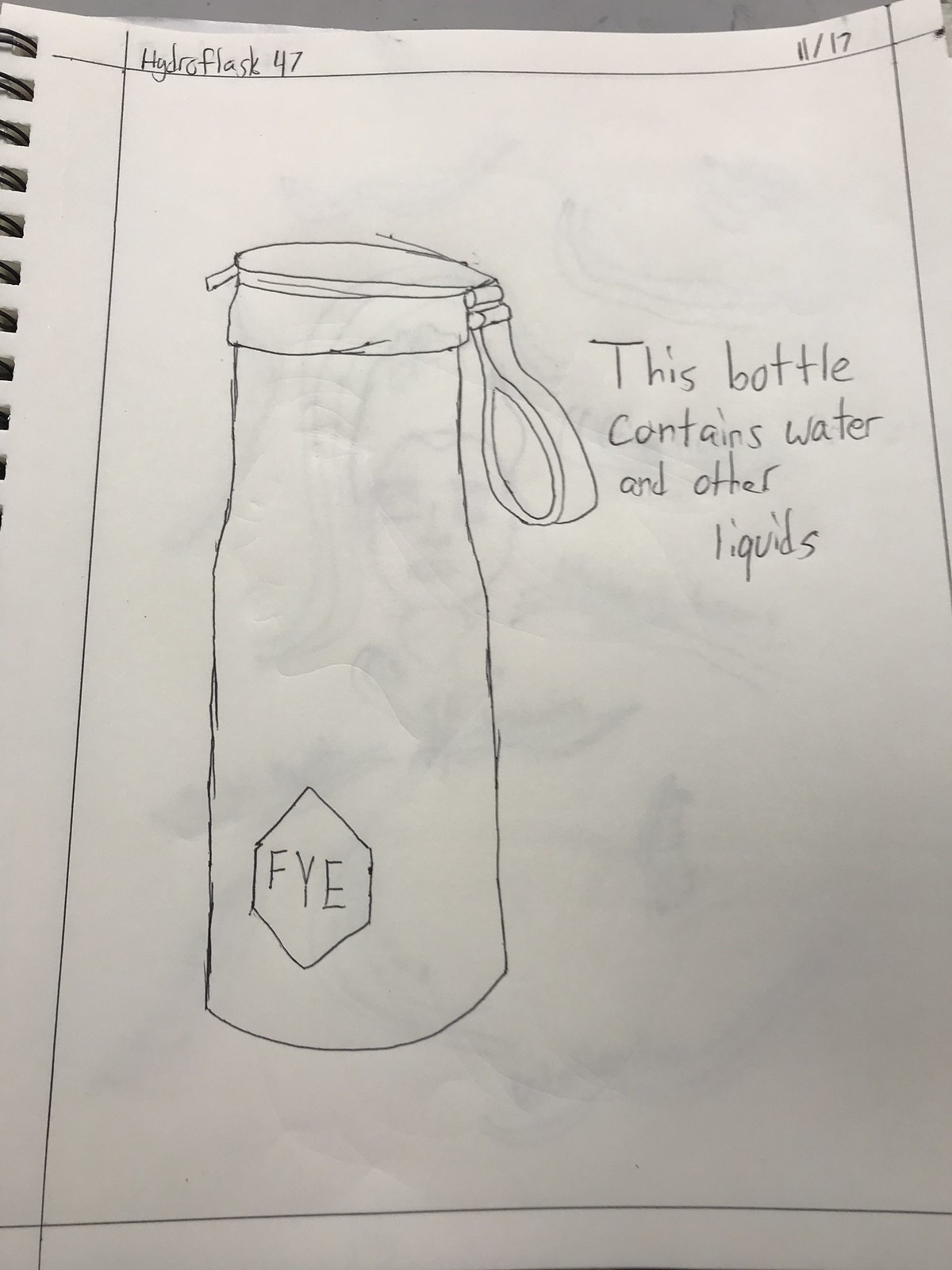This is a color photograph of a drawing on a white sketchbook page, featuring a simplistic, black and white outline of a Hydro Flask reusable water bottle. The sketch is executed in pen, emphasizing its rudimentary style. The bottle, resembling a tall, vertical cylinder, includes a cap and a carrying strap hanging from the right side of the cap. An octagonal shape near the bottom of the bottle contains the letters "FYE." To the right of the bottle, aligned with the strap, is a handwritten note stating, "this bottle contains water and other liquids." Above the drawing, in the upper left corner, it is labeled "Hydro Flask 47," and in the upper right corner, "8/17." Black spiral binding is visible on the left side, more prominently in the upper half. There is also some bleed-through from another drawing on the reverse side of the page, which appears to include the faint image of a person's face and other ambiguous shapes.